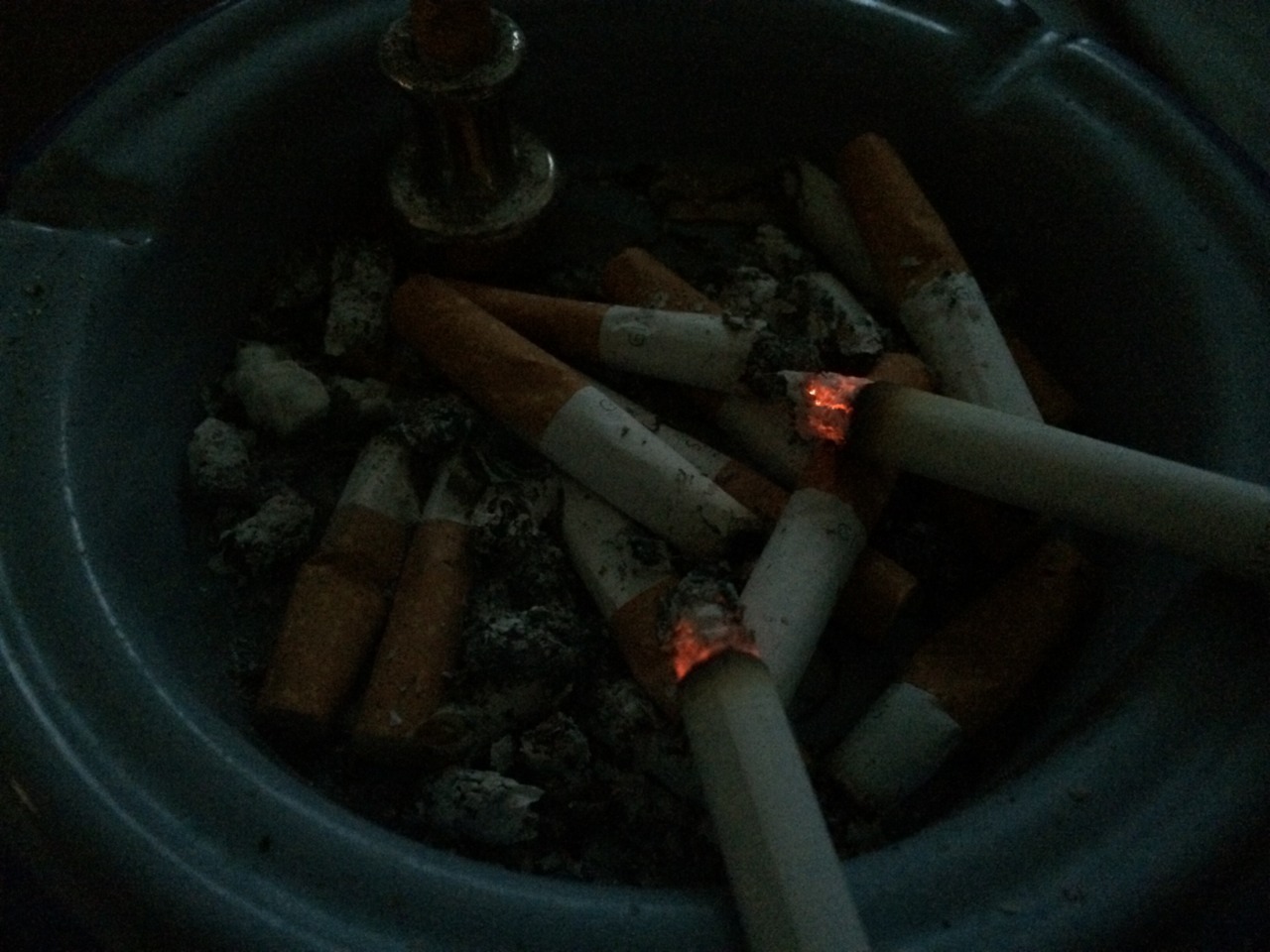This dimly lit photograph features a close-up of a small, teal ceramic ashtray with white and blue outlines at the edges. The ashtray is filled with numerous cigarette butts and piles of ashes, indicating heavy use. In the middle of the ashtray, there is a mix of fully smoked and half-smoked cigarettes, all of which are white with brown filters. Notably, two cigarettes, positioned at the top right corner, are still lit, their orange embers casting a slight glow. Additionally, there is a small gold object situated at the top left side within the ashtray. The overall dark ambiance of the image enhances the focus on the details of the ashtray and its contents.